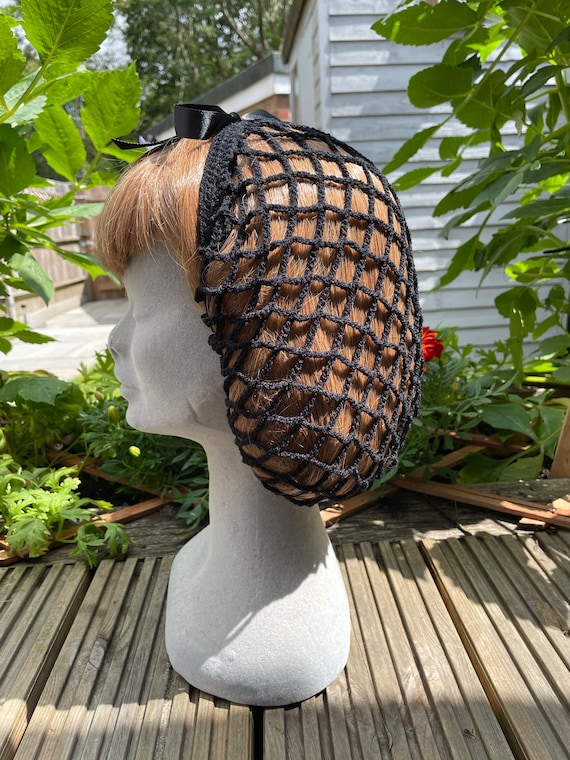In this bright, daytime color photograph, the scene is set outdoors on a wooden deck with corrugated planks. A prominent white facial mannequin bust, featuring sculpted shoulders, is the central subject. The mannequin is turned slightly to the left, donning a tan, reddish-brown wig with bangs. The hair is neatly gathered and secured in a bun at the back of the head, encased in a black crocheted snood adorned with a black satin bow. The snood, with its open square weave, highlights the craftsmanship of the crocheted thread.

In the background stands a house with gray siding and a two-way roof, adding a residential feel to the composition. Behind a wooden fence and a possibly concrete driveway, lush foliage and verdant trees further enhance the tranquil setting. The overall style suggests a blend of photographic representationalism and product photography, meticulously capturing the detailed accessory within a realistic environment.